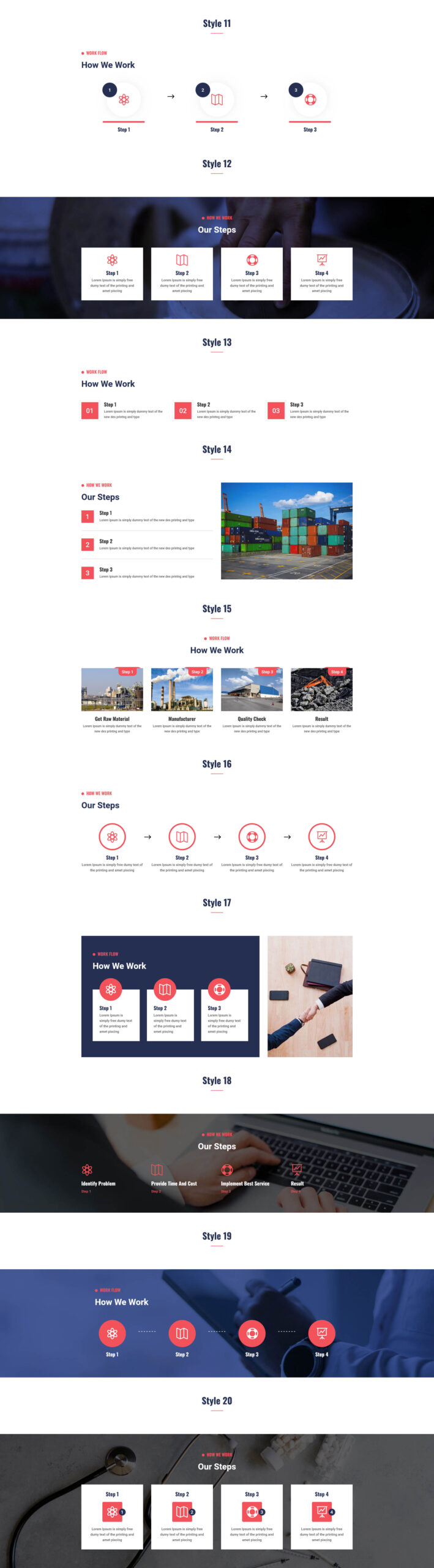The image depicts a compressed screenshot of a website layout template. At the top center, the text "Style 11" is prominently displayed. Directly beneath, there's a blue banner divided into four segments. Above this banner, the text "Step 12, Style 12" is visible. Positioned between the "Style 11" and "Style 12" sections are three blocks set against a white background. The first block is labeled "How We Work," while the second and third blocks, titled "Step 2" and "Step 3" respectively, lack additional titles.

Below this series of steps, another banner labeled "Style 13" is visible, reiterating "How We Work," suggesting these may be stylistic options for a website. Further down, various styles are enumerated, from "Style 16" to "Style 20," indicating different layout choices available for the website design.